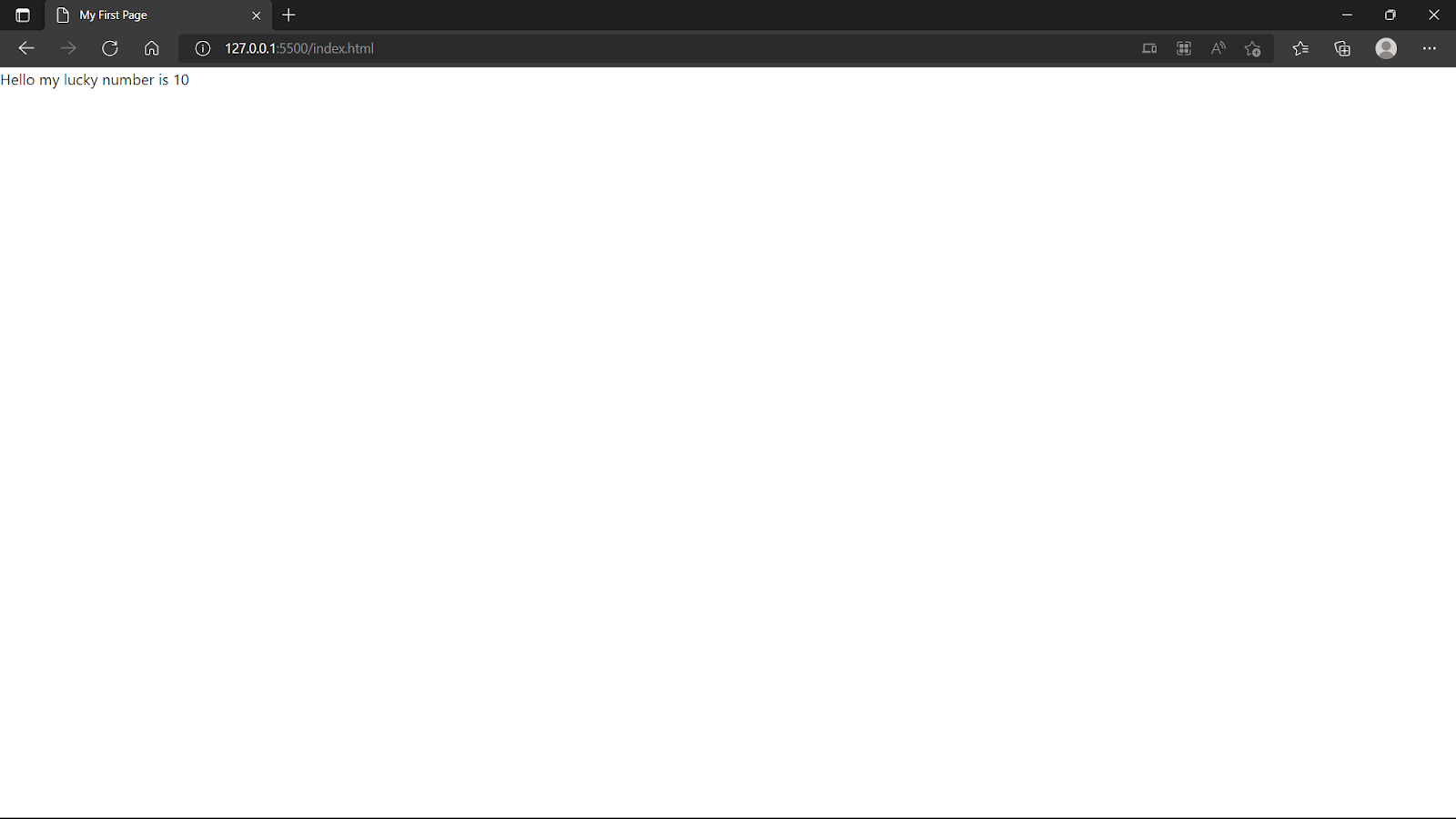Screenshot of a Beginner's Web Page Creation Interface

The screenshot appears to depict a web page creation interface, likely for a user constructing their very first web page. The interface features a prominent black bar at the top, which contains various navigational and functional icons. 

In the upper left-hand corner of the black bar, there is a logo, though its specifics are difficult to discern. To the right of the logo is the text "My First Page," indicating the title of the created webpage. Adjacent to this text, there are icons to exit the page and add additional elements. 

On the far right side of the black bar, there are three familiar window control buttons: minimize, maximize/expand, and exit. Beneath this top bar, there is a standard navigation toolbar featuring back and forward arrows (with the back arrow currently active), a refresh button, a home icon, and an information button. There is also a label displaying "T27001," likely an identifier for the current session or page.

Further to the right extends a row of gray icons, which are somewhat indistinguishable. Among them, there seems to be an option to star the page, add a screen, and an icon suggesting user profile customization. At the far right end of this row is a button represented by three dots, typically used to indicate additional settings or options.

The central white space of the interface displays the text "Hello, my lucky number is 10," written in a gray font. This message appears somewhat peculiar and may be a placeholder or user-added content.

Overall, the screenshot provides a glimpse into a basic web page creation tool, highlighted by its user-friendly icons and navigation aids.